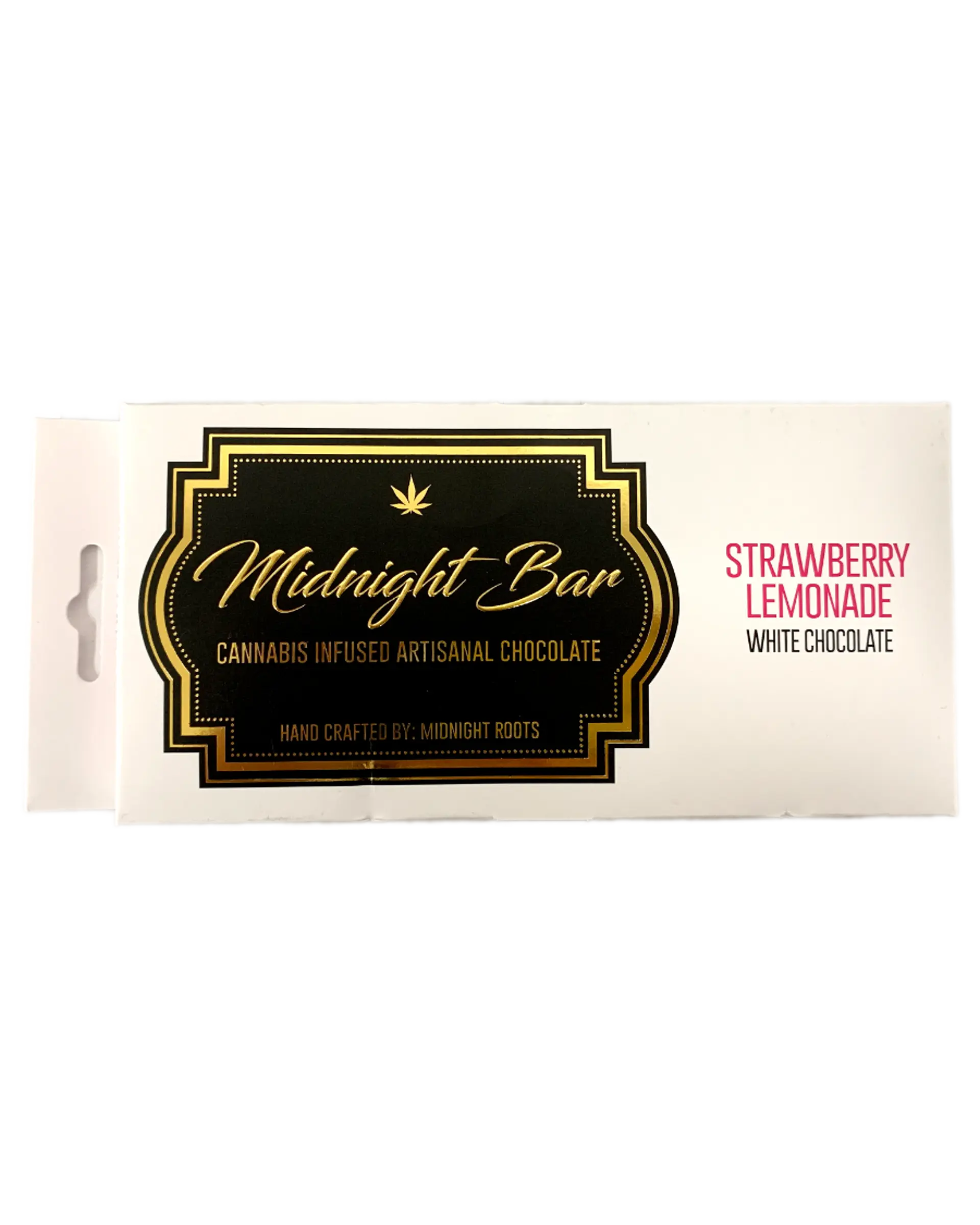This photograph showcases an elegant and meticulously designed cannabis packaging. The packaging features a striking contrast between its elements; one side of the image displays a pale pink background, while the other side highlights an Art Deco-inspired graphic. The graphic is set against a black background, accentuated by a sophisticated gold outline and gold font, exuding a luxurious aura. At the top of the black section, a gold cannabis leaf stands prominently, adding a touch of opulence.

The central text in gold font reads, "Midnight Bar," indicating that this is a cannabis-infused artisanal chocolate crafted by Midnight Roots. Adjacent to this, in eye-catching pink font, it announces the flavor variant: "Strawberry Lemonade." Below, in black font, it specifies the type of chocolate as "White Chocolate."

The top of the packaging features a cutout, designed for hanging the product on a retail shelf. This appears to be a high-quality cardboard package, evidenced by subtle shadowing and light reflections that give it a three-dimensional feel. The image itself is of exceptional quality, crystal clear, and allows all text to be easily readable, highlighting both the craftsmanship of the packaging and the skill of the photographer.